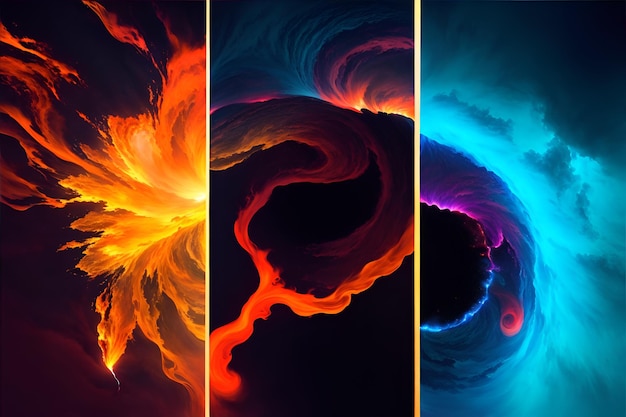This three-part abstract illustration, evenly divided into thirds, captures a mesmerizing display of vivid colors and dynamic forms against a deep, dark background. In the first section, a fiery, reddish-orange cloud erupts dramatically from the side, set amidst a stark black backdrop with subtle stripes. The central image showcases a lava-like flow over a dark mass, which billows into a captivating cloud of multicolored smoke featuring hues of purple, red, gold, and blue, enhanced by a faint purple glow. In the rightmost section, a swirling sky combines shades of azure and teal with a black mass on the left, emitting swirling purple and blue smoke interspersed with small red swirls and a reddish circle. This visually stunning triptych is tied together by the recurring presence of a black element in each segment, creating a cohesive yet dynamic blend of colors and forms.